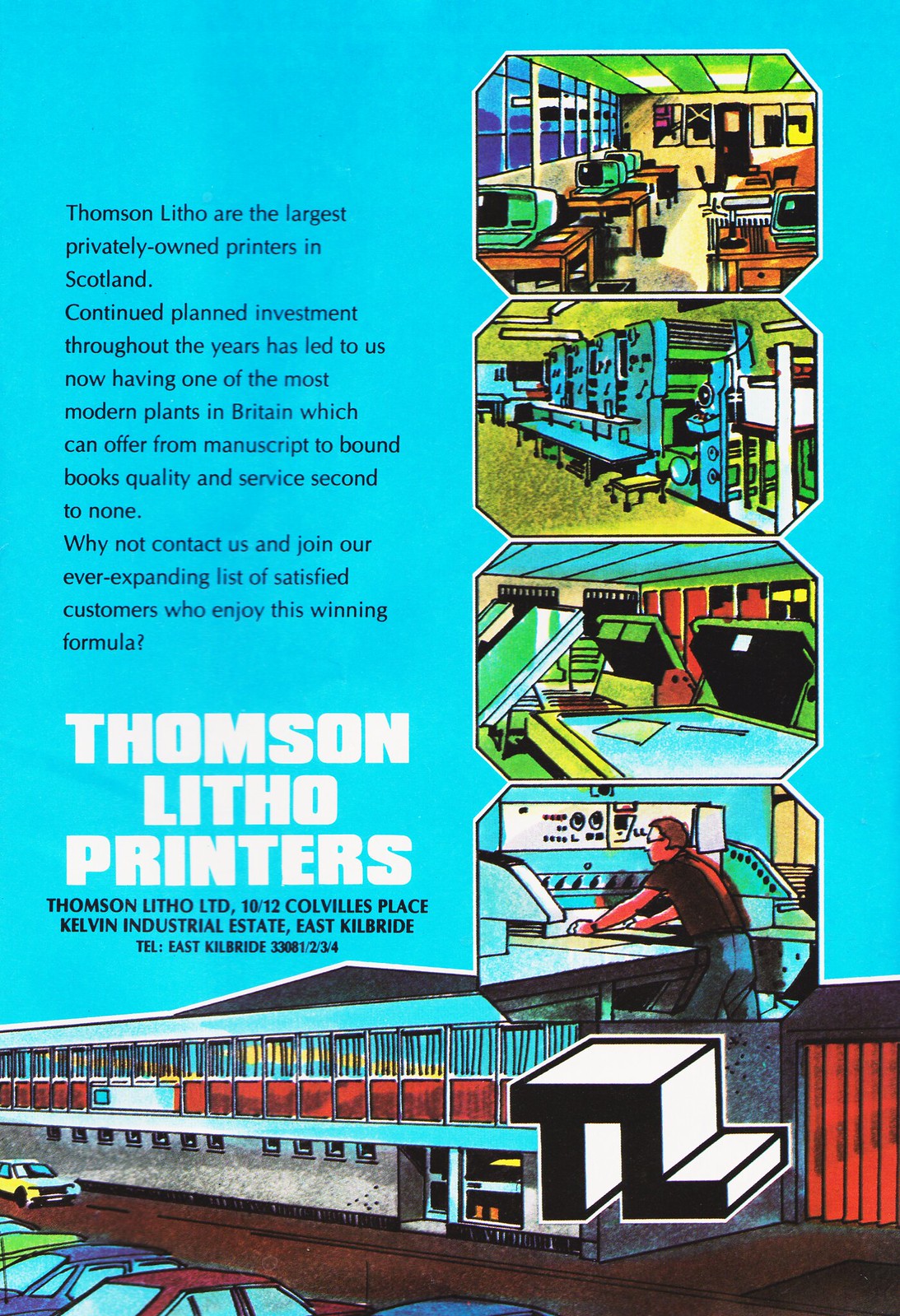The image is a vivid advertisement for Thompson Litho printers, prominently displayed on a bright neon blue letter-sized sheet. The portrait-oriented ad is rich in color, featuring an array of primary tones such as greens, blues, and reds with marker or watercolor-like illustrations lending it a retro feel. Dominating the left side is a well-crafted text that states: "Thompson Litho are the largest privately owned printers in Scotland. Continued planned investment throughout the years has led us to now having one of the most modern plants in Britain, which can offer from manuscript to bound books, quality and service second to none. Why not contact us and join our ever-expanding list of satisfied customers who enjoy this winning formula?" 

On the right side, several illustrations show the various facets of the printing plant, including a computer lab, a state-of-the-art printing press featuring four machines, and a section with drawing tablets or editing monitors. At the bottom of the sheet, another larger illustration depicts the exterior of the plant, complete with parked cars, a blue and black building with red paneling, and a red corrugated metal door.

The ad is finished with the company logo and their contact information: "Thompson Litho LTD, 10-12 Colesville's Place, Kelvin Industrial Estate, East Kilbride," alongside their telephone number in a large white all-caps font. Overall, this vibrant and detailed composition captures the extent of Thompson Litho's capabilities and their modern facilities, inviting potential customers to join their growing list of satisfied clients.